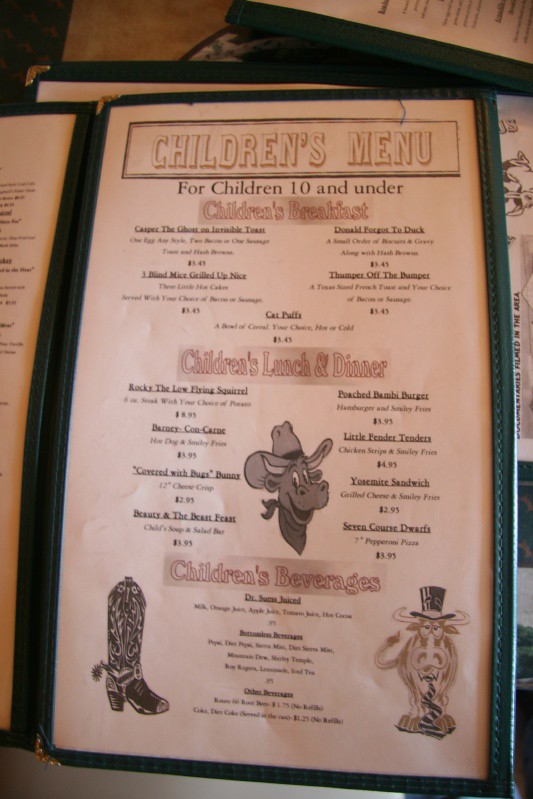This is a photograph of a children's menu presented inside a sleek black folder. The menu page itself has an ivory background, giving it a nostalgic, rustic charm. The text is styled in an Old West script, with "Children's Menu" prominently displayed at the top, followed by a note indicating it's for children aged 10 and under. Categories such as "Children's Breakfast," "Children's Lunch and Dinner," and "Children's Beverages" are highlighted in red, contrasting with the rest of the black text. 

Illustrations add a playful touch to the menu: a cowboy boot with a spur decorates the lower left corner, while the right side features an amusing image of a cow or bull dressed in a top hat and tie. Centrally positioned is a charming bull adorned with a cowboy hat and a small kerchief around its neck. 

The text detailing the menu items is notably small, making it difficult to read, but the overall presentation suggests a whimsical, kid-friendly dining experience. The menu appears to be open and resting atop a collection of other menus.